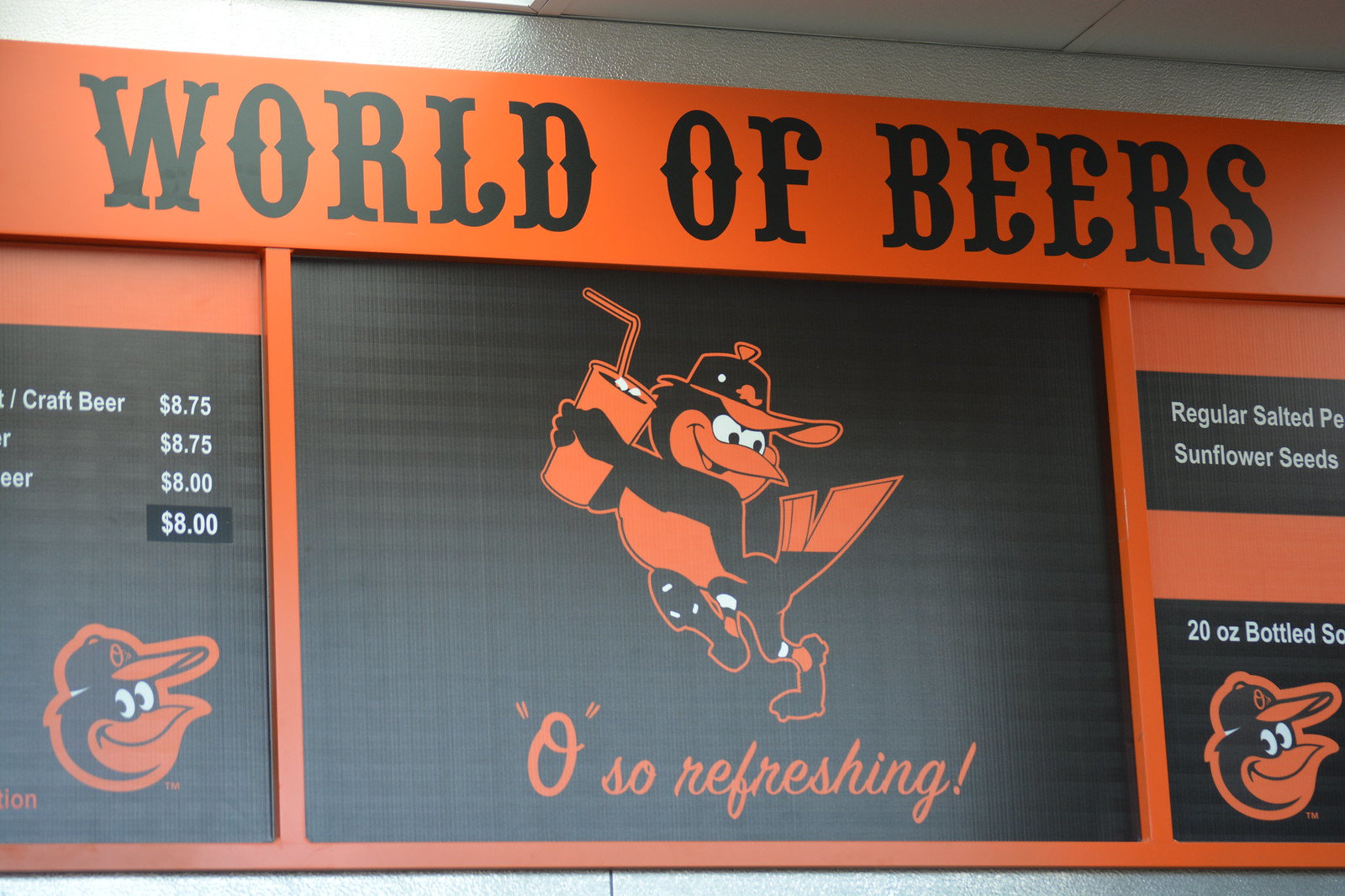The image depicts a colorful menu board for a restaurant or concession stand called "World of Beers." The board is primarily orange with black lettering, and the backdrop is wooden. Dominating the center of the image is a cartoon depiction of a bird, likely the mascot for the Orioles baseball team, wearing a cap and holding a cup with a drink. This animated bird exclaims "Oh So Refreshing" in bold, accompanying the drink it's holding. At the top of the board, "World of Beers" is prominently displayed in black letters on an orange banner.

The menu features pricing for various items, though some details are partially cut off. Clearly visible is a craft beer priced at $8.75 and other items, such as regular salted peanuts, sunflower seeds, and a 20-ounce bottled soda. The board's appealing colors and playful mascot suggest it might be found indoors at a baseball stadium, potentially near a concession area where snacks and beverages are sold.